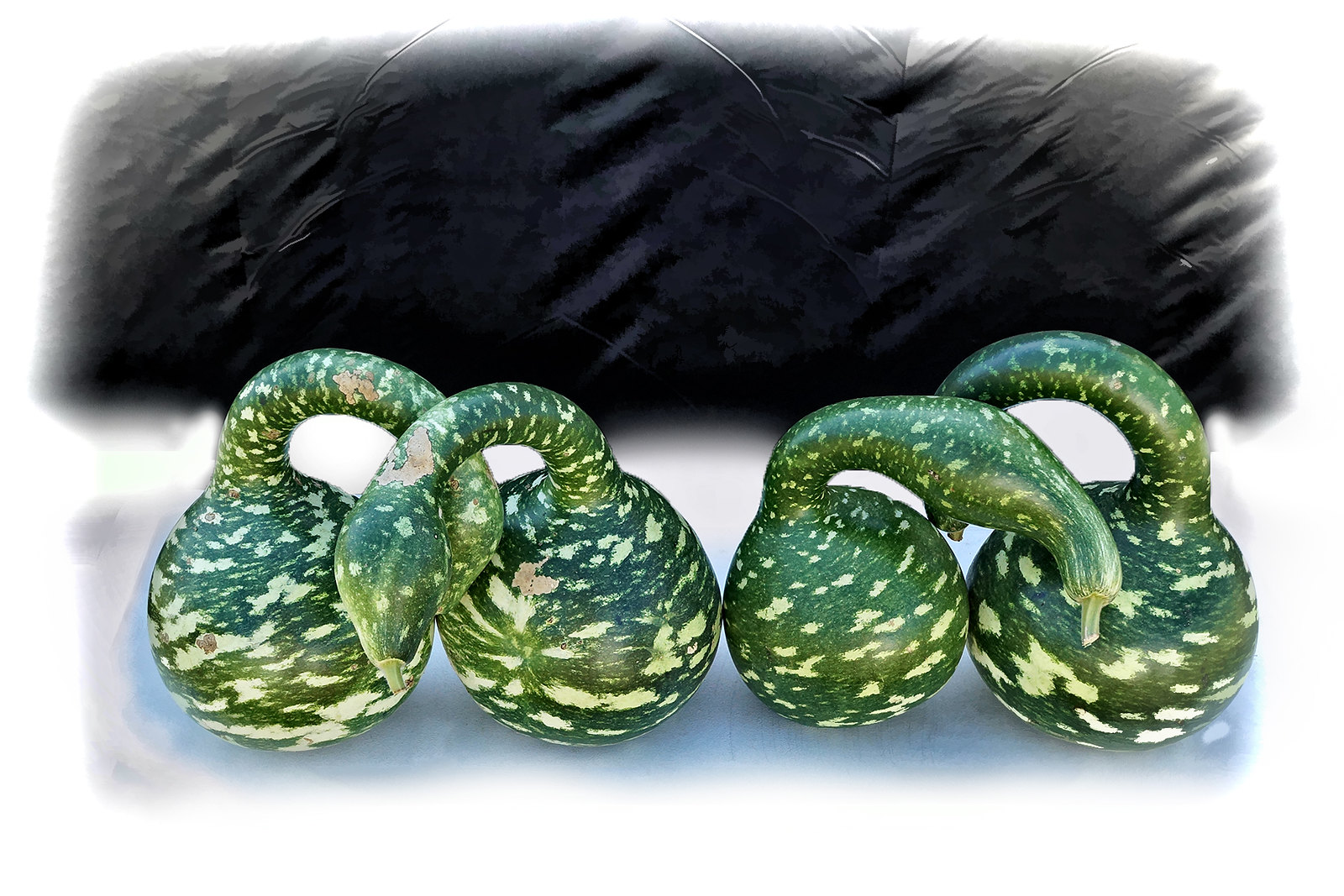The image depicts four unique green gourds, each adorned with yellow and white spots. These gourds are round at the base with long, bulbous stems that elegantly curve and extend to the side, almost resembling the elongated necks of swans or ducks nestled together. They convey an impression of intertwined creatures due to their intriguing positioning. The gourds rest on a blue cloth, with a backdrop of black fabric that displays visible wrinkles, suggesting a soft texture. The arrangement of these unusual gourds on the blue and black fabrics creates a striking contrast, highlighting their vibrant green hue and distinctive shapes.